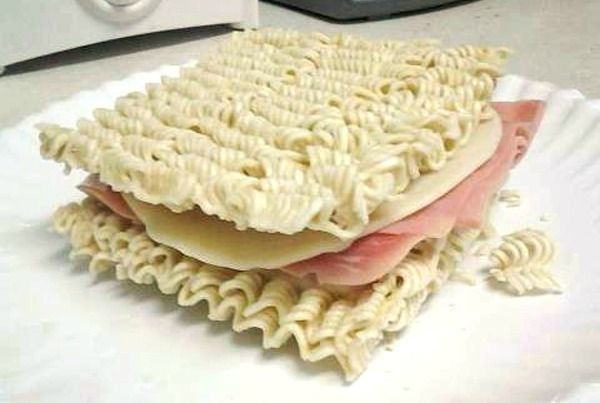The image depicts an unconventional sandwich made with two squares of uncooked ramen noodles serving as the "bread." Sandwiched between the crispy ramen squares is a slice of circular, white cheese, likely provolone due to its lack of holes, placed directly beneath the top ramen square. Below the cheese, there are thin slices of ham, adding a hint of pink color and texture contrast to the creation. This ramen sandwich is perfectly centered on a white paper plate, which rests on a kitchen counter that features a white surface speckled with black. Although slightly obscured, some kitchen accessories are visible in the background, suggesting this is a home kitchen setting. The counter space enhances the homely feel of the scene, completing the peculiar yet intriguing culinary setup.